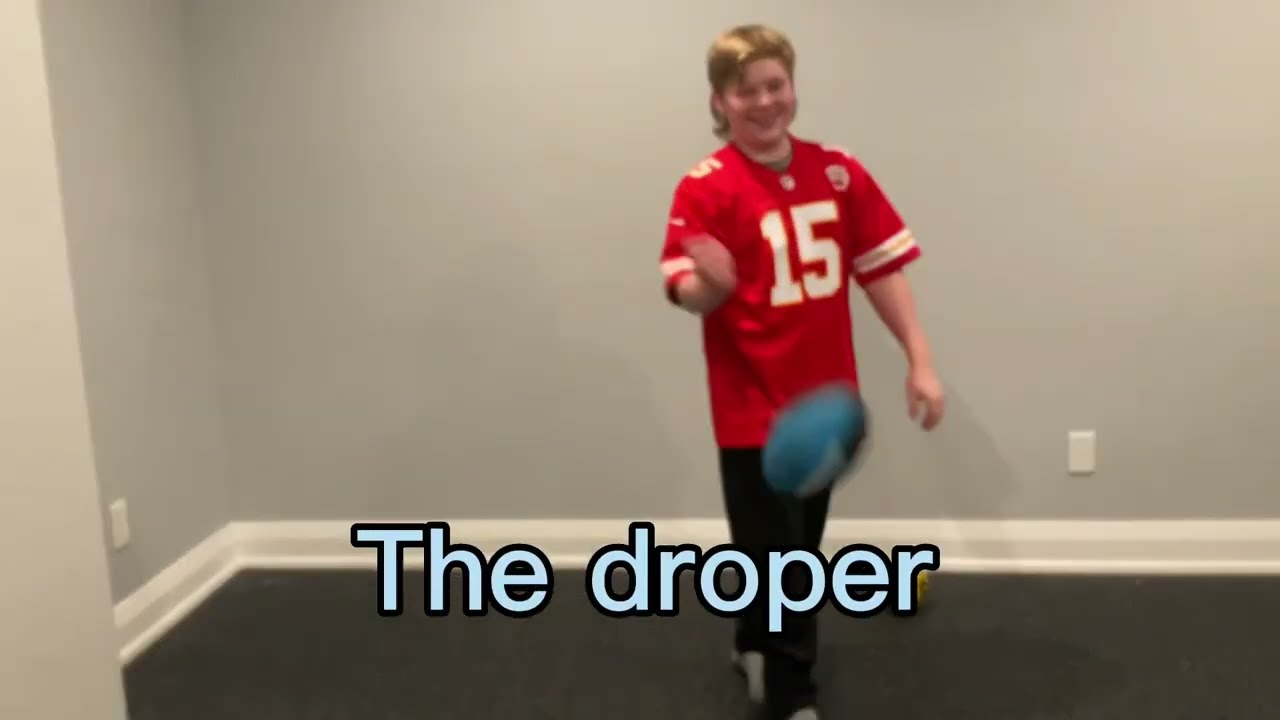The image is a somewhat blurry indoor photograph, likely taken with a smartphone, depicting a young boy, approximately 14 years old, with blond, medium-length, well-groomed hair, smiling broadly. He is clad in a red football jersey with the number 15 in white, complemented by white and gold stripes on its short sleeves, and black pants. The boy appears to be in mid-motion, seemingly drop-kicking a football, although it’s unclear if contact has been made. The football is an unusual greenish or aqua color and shows signs of rotation or motion blur.

Set in a barren room with gray drywall, white base molding, and a dark gray carpet, the image also features a bit of a white door frame on the left side and a peculiar covered outlet near the bottom right. Centered at the bottom in light blue text with a black border, the caption reads "Droper" (spelled D-R-O-P-E-R), adding a mysterious element to the otherwise straightforward scene.